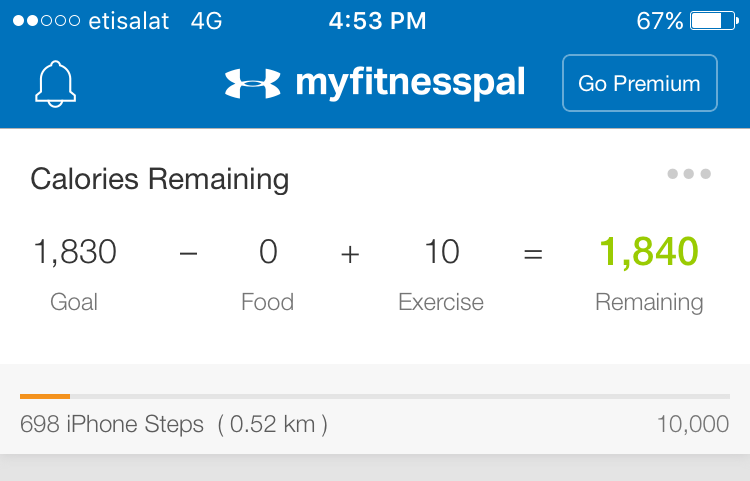The top of the image features a dark blue background with a white circle and three blue circles, displaying the text "ETISALAT 4G." The top right corner shows the time 4:53 PM, a battery icon at 67%, and a notification bell. Below that, there is an Under Armour logo followed by the text "MyFitnessPal" and a button labeled "Go Premium."

The main portion of the image has a white background. It displays "Calories Remaining" with a goal of 1,830 calories. No calories from food are subtracted, and an additional 10 calories are added from exercise, leaving a total of 1,840 calories remaining, highlighted in green. Above this section, there's a horizontal ellipsis. 

Below this, a gray box features a two-tone progress bar: an orange line transitioning into a gray line, indicating "698 iPhone steps" which is approximately "0.52 KM" out of a goal of "10,000 steps."